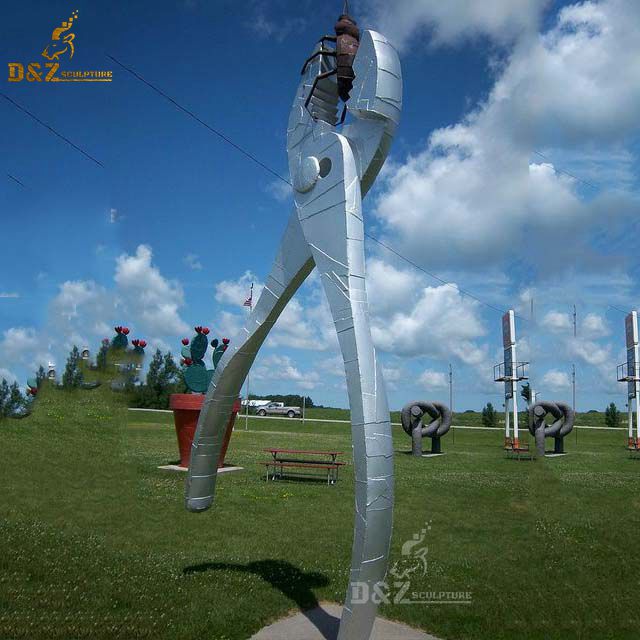This image features a captivating outdoor art exhibit set against a backdrop of a blue, cloud-filled sky and a lush green landscape, dotted with trees in the distance. In the foreground stands an oversized, 20-foot-tall silver wrench sculpture, balanced dynamically on one of its prongs with the other extending into the air. Clamped within the wrench is a black insect, resembling an ant. Centered behind this striking piece, a red flower pot with green cactus plants adorned with tiny red flowers adds a vibrant contrast. To the right of the wrench, a wooden bench sits invitingly, offering a place for viewers to rest. Further to the right are intriguing silver and grey metal sculptures that spiral upwards into circular forms, adding an abstract element to the scene. All the sculptures are anchored on concrete slabs, surrounded by manicured green grass, integrating seamlessly into the natural park-like setting. The image also contains faint text details in the top left and bottom left corners.